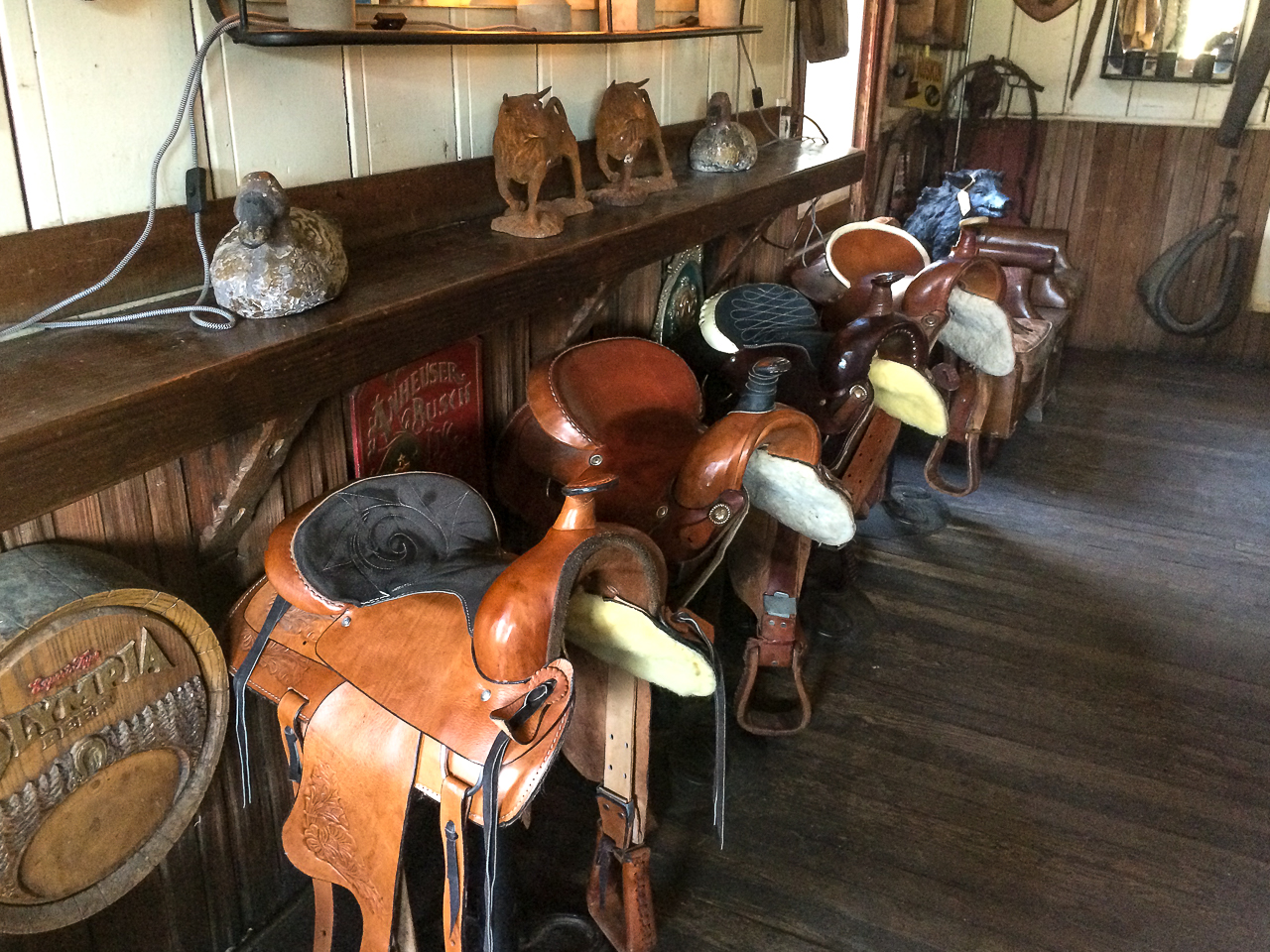The image showcases a rustic barn or house interior, lined with a row of horse saddles mounted next to a wooden counter. The setting exudes a rugged, vintage charm with all furnishings predominantly made of wood. The saddles, positioned along the wall, boast a variety of designs and materials, including black bases and ornate leather finishes, highlighting their worn but intricate craftsmanship. Behind the saddles, the wooden wall extends up to a halfway point before transitioning to a white upper section. Below the counter, there are several old, rustic signs, contributing to the antique ambiance.

On the wooden countertop, a couple of duck and wolf figurines stand out, intricately placed in pairs. To the left at the base of the counter, there is a round wooden container affixed to the wall, adding to the room's rustic aesthetic. As the eye moves to the upper right, two leather chairs can be seen behind the saddles, and in the distant corner, a figure resembling a javelina, possibly stuffed or metal, adds a unique focal point. The flooring consists of narrow, small wooden planks, enhancing the overall wooden theme of the interior. Scattered barn equipment and possibly traps or snares further emphasize the rural vibe. This scene might well be a store of antiques, filled with historical and rustic memorabilia.